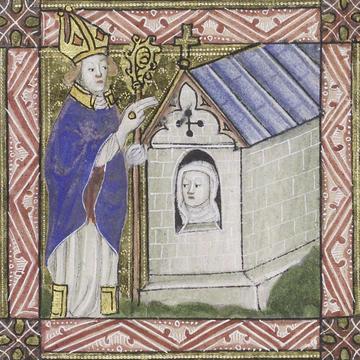This image appears to be a photograph of a painting or stained glass window, likely from the Renaissance period or Middle Ages. It features a religious figure, possibly a Catholic bishop or priest, adorned in a blue cloak with a white robe trimmed in gold. The figure is wearing an ornate, triangular, golden mitre hat and holding a gold scepter, and raises his right arm in benediction. Surrounding this central figure is an intricate border composed of mauve and beige diagonal lines. Inside the scene, there is a small mausoleum-like structure or miniature church made of white bricks with a gray roof and a crucifix atop it. Within this structure is what appears to be a white marble statue or bust of a woman. The vivid colors such as various shades of blue and meticulous details suggest the medium might be stained glass, capturing a religious ritual or symbolic blessing from the historical context. The overall imagery reflects rich religious iconography, indicative of early European art.